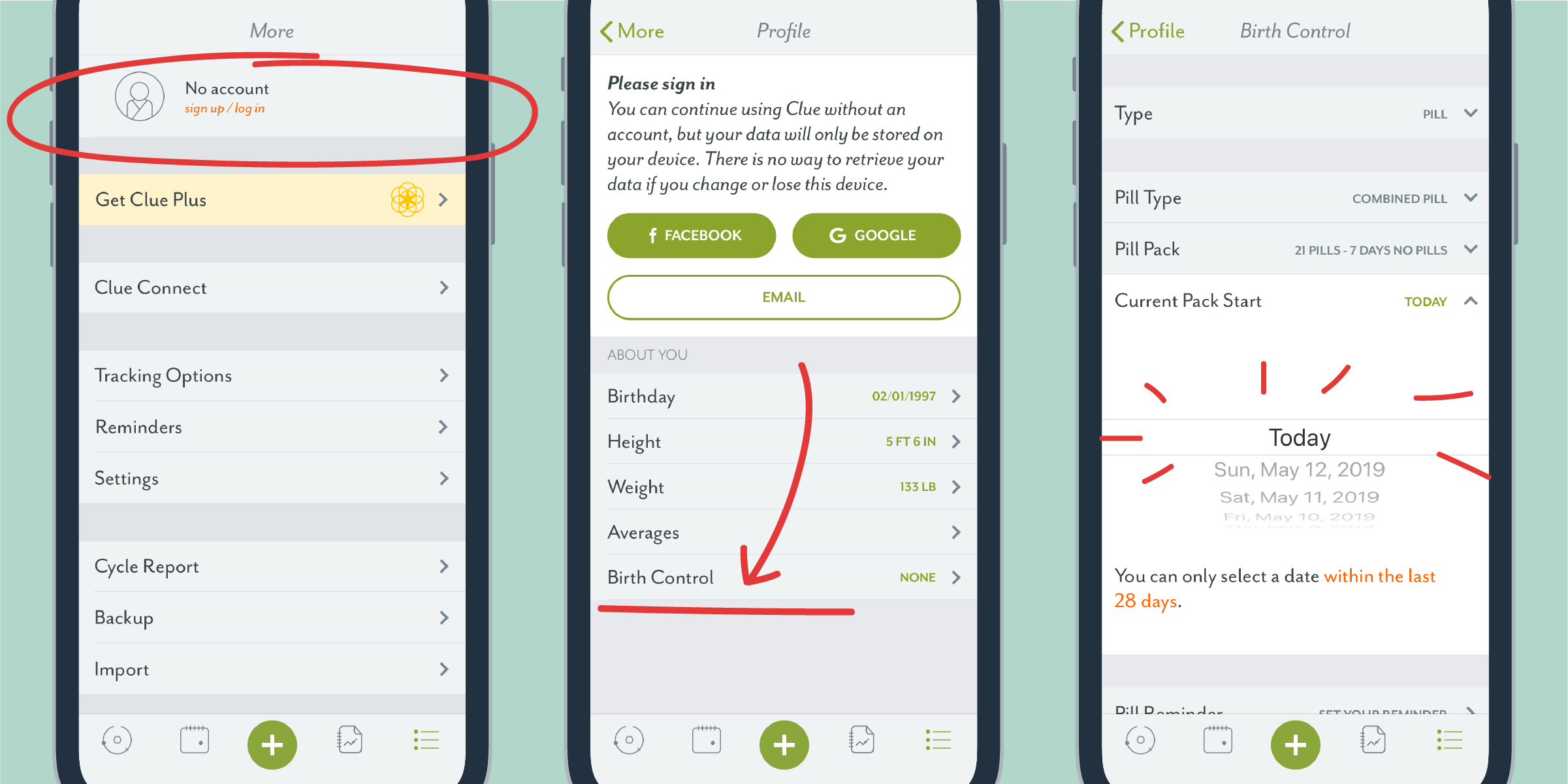The image consists of a series of app screenshots captured on a smartphone, presented in a step-by-step sequence from left to right. The first screenshot features the app's welcome screen, where the word "More" is displayed at the top. Below, the message "No Account" is prominently circled in red, drawing attention to the options "Sign Up" or "Log In." The next screenshot transitions to the profile page, which prompts the user to sign in. Here, there are multiple sign-in options: Facebook, Google, or Email. Additionally, a red arrow at the bottom directs attention towards a menu item labeled "Birth Control." 

The final screenshot focuses on the "Birth Control" section, with the term "Birth Control" clearly displayed at the top. The word "Today" is encircled with red lines resembling a spark effect, indicating the user's action. This screen provides a message noting that users can only select a date within the last 28 days. It also mentions "Current Start Pack Today," indicating that the user is initiating their birth control regimen. This sequence of images seems to illustrate how the app assists users in managing their birth control, suggesting it may be geared towards birth control awareness and management.